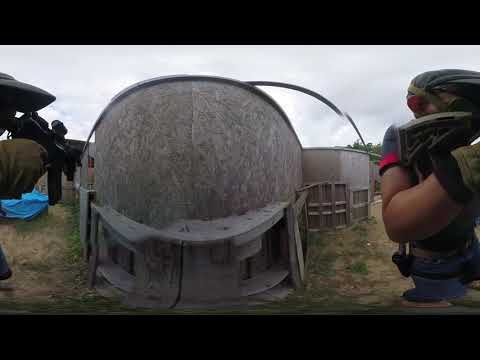In the foreground to the right, a person dressed in a short-sleeved shirt, blue jeans, a black gear belt with additional bullet packages, a safety helmet, and a glove is prominently featured holding an automatic rifle. This individual is standing next to a large gray dome-like structure attached to a gray building, which may serve as a storage area for ammunition or guns. To the left, a blue tarp lies on the dry ground, which is interspersed with patches of green grass and weeds. The setting is a shooting range, where a less visible second shooter can be seen holding their rifle and aiming in a different direction. The background is forested, providing a natural backdrop to the scene. The overall ground is a mix of brown patches and green vegetation, and the sky above is predominantly white and cloudy, suggesting an overcast day.